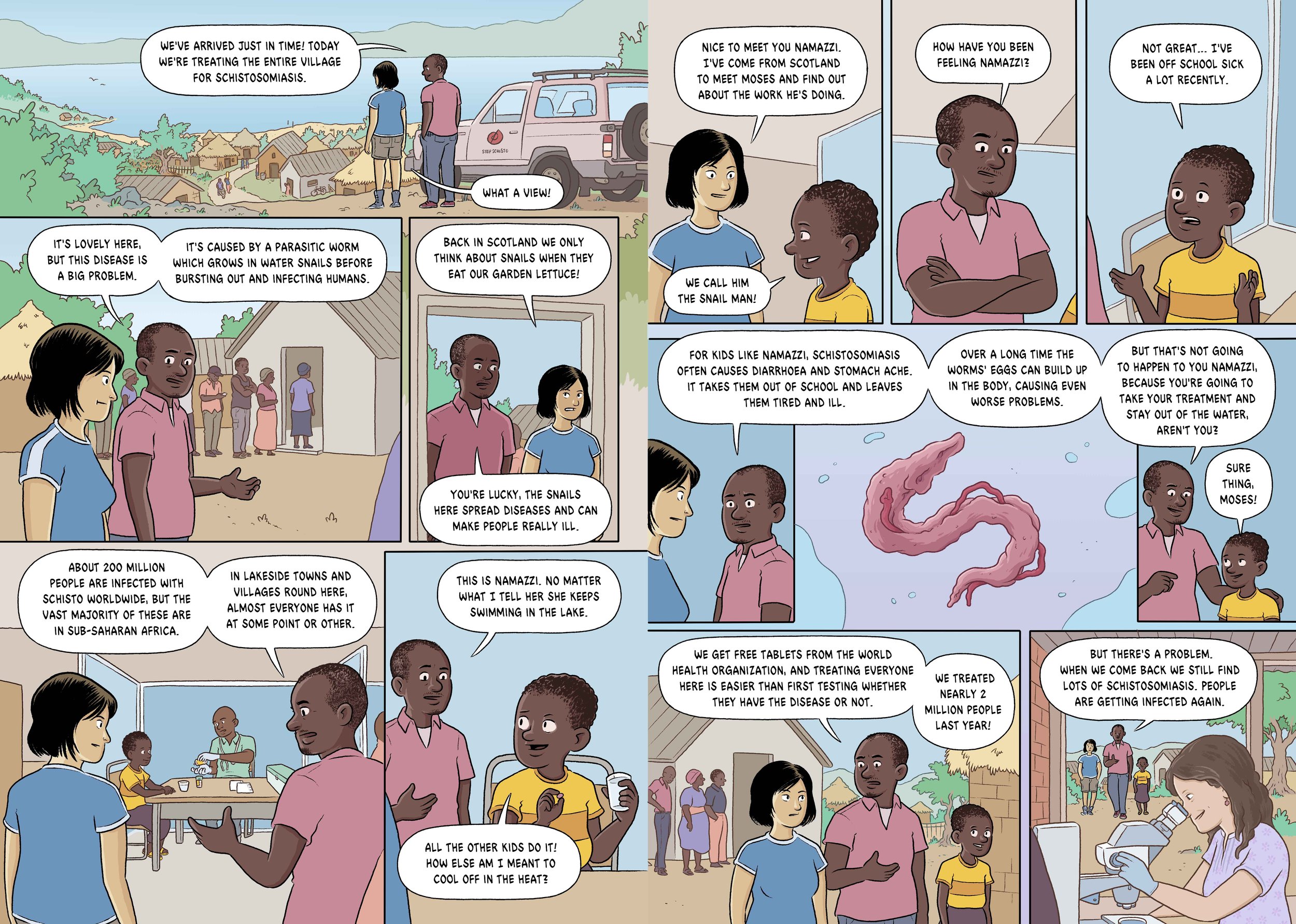The image is a detailed cartoon composed of multiple comic book panels. The narrative features three distinct characters: a black man in a red shirt, an Asian woman with short brown hair in a blue shirt, and a young black boy wearing a yellow shirt with a single darker yellow stripe across the chest. In the first panel, the man and the woman are overlooking a scenic village by a lake, where the man states, "We've arrived just in time. Today we're treating the entire village for schistosomiasis." The woman responds, "What a view." 

Subsequent panels introduce more context, revealing that they are in an African country and explaining the impact of schistosomiasis, a disease caused by parasitic worms that grow in water snails. The man, referred to as "the snail man," has come from Scotland to collaborate with a local named Moses. They work to combat the disease, which causes diarrhea, stomach ache, and fatigue in children like Namazi, keeping them out of school and impacting their overall health. The cartoon emphasizes the importance of treatment and avoiding contaminated water to prevent severe complications from the parasite buildup over time. The characters are depicted engaging with the community and educating them on the necessary precautions and treatments.